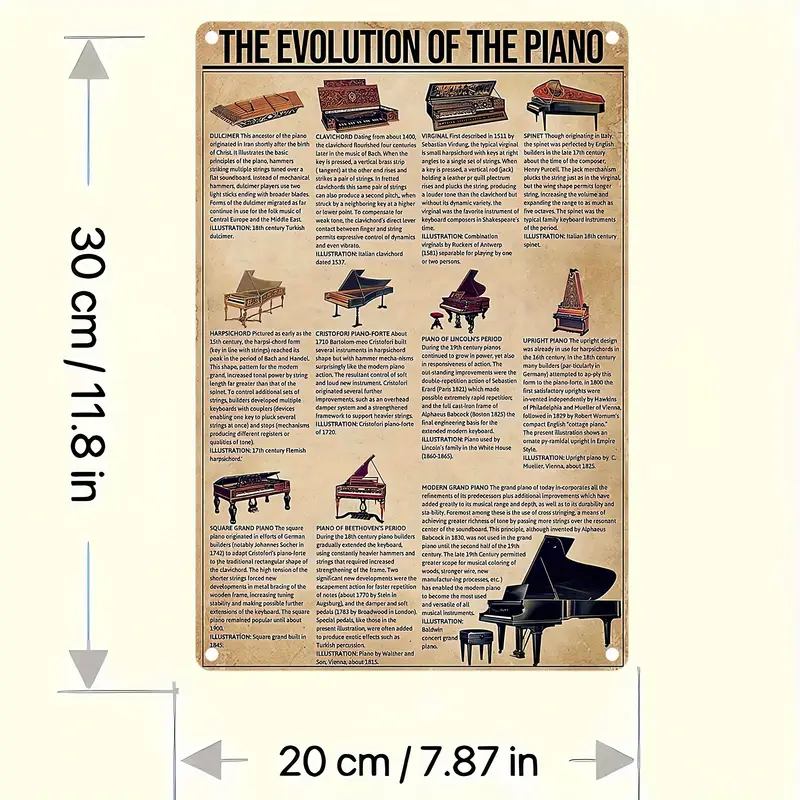The image showcases a large square poster against an ivory or pale yellow background. The poster, vertically oriented and likely made of metal, has a light brown color with a title at the top that reads "THE EVOLUTION OF THE PIANO" in bold black uppercase letters. Below the title, the poster is divided into three sections, each illustrating the historical progression of pianos. 

The top section features four small images of different pianos, each with a descriptive paragraph beneath it, aligned to the left. The middle section also consists of four images with accompanying text. The bottom section is slightly different: the left side contains two smaller images with paragraphs, while the right side prominently displays a larger illustration of a black grand piano with its hood open, accompanied by a paragraph situated partly above and to the side of the piano. 

Measurements are provided along the sides of the poster: vertically on the left, "30 CM / 11.8 IN" is printed with arrows indicating up and down, while horizontally at the bottom, "20 CM / 7.87 IN" is noted with arrows pointing left and right. The poster offers a detailed visual and textual history of the piano through eleven different images, including representations of instruments such as the harpsichord, square grand piano, and upright piano.